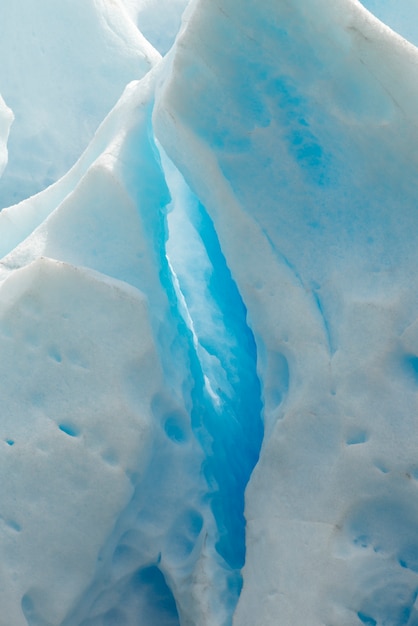This detailed image features a very zoomed-in view, showcasing a mass of ice that resembles a glacier, potentially captured in an outdoor Antarctic landscape. However, with the high level of zoom, it could just as easily be part of someone's freezer. The scene includes a range of colors, primarily whites and off-whites, transitioning into light blue shades and culminating in very dark blues. The light blue and white hues dominate the center of the photo, creating a streaking effect from the top left to the bottom right. The composition is well-centered and decently symmetrical, with the focal point resting in the middle. There are no text or words on the image, allowing the intricate details of the ice to stand out against the surrounding off-white and blue tones.